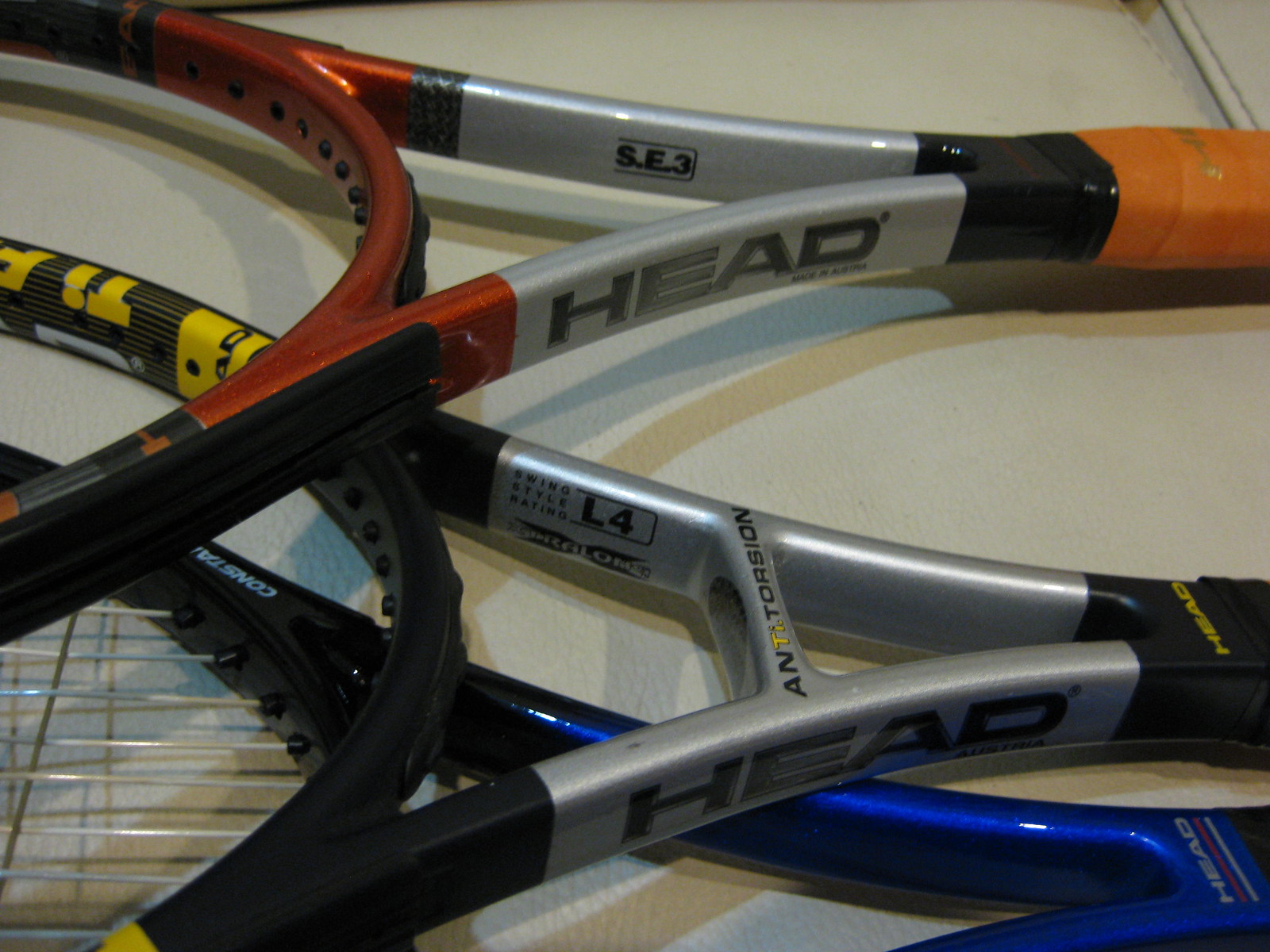This detailed image captures a close-up of the yoke areas of three tennis rackets where the oval head meets the handle grip. The rackets are stacked on top of one another, and the photo focuses on their necks and grips, providing a clear view of the brand and specific details. The topmost racket features a medium shade of orange handle grip with an orange and silver frame, and displays the word "HEAD" in black letters and "SE3" markings. The middle racket has a silver frame with black detailing, including a black grip and yellow lettering spelling "ANTI-TORSION" with the "TI" highlighted in bright fluorescent yellow. It also features a rating of L4 for swing style. The third racket at the bottom is a striking royal blue, possessing a metallic sheen, and is the only one that still has strings. All three are placed on a flat surface, which could either be a beige countertop or possibly a leather material. The brand "HEAD" is prominently displayed on all rackets, signaling their make and reinforcing the sporting context of the image.